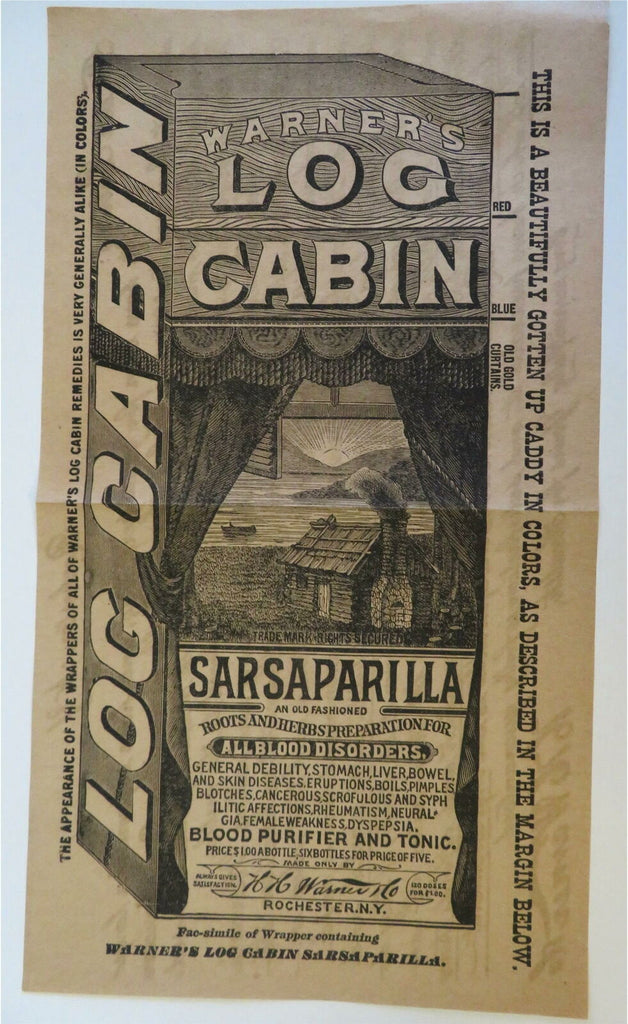This is a detailed photograph of an old-fashioned advertisement, likely from a newspaper and resembling a vertical fold-out page. The advertisement is monochromatic, entirely in black and white, set against a vintage, slightly creased brown paper background indicative of age. At the top, the advertisement prominently features the heading "Warner's Log Cabin." Beneath this title, there is an intricate sketch depicting a quaint log cabin with smoke billowing from its chimney. In this picturesque scene, the sun rises over a mountain, illuminating a lake with a boat on its waters, which adds to the rustic charm.

The text below the illustration reads "Sarsaparilla, roots and herbs, preparation for all blood disorders," emphasizing the ad's focus on a medicinal tonic. It further promotes the product as a "blood purifier and tonic," suggesting it could address issues related to the stomach, liver, bowel, and skin, thus highlighting its broad medicinal claims. The fine print on the sides adds that the appearance of the wrappers of all Warner's Log Cabin remedies is notably similar in color, which is an ironic note given the black-and-white composition of the ad. This advertisement embodies the nostalgia of a bygone era, perhaps from the 1800s, when such tonics were common household items.